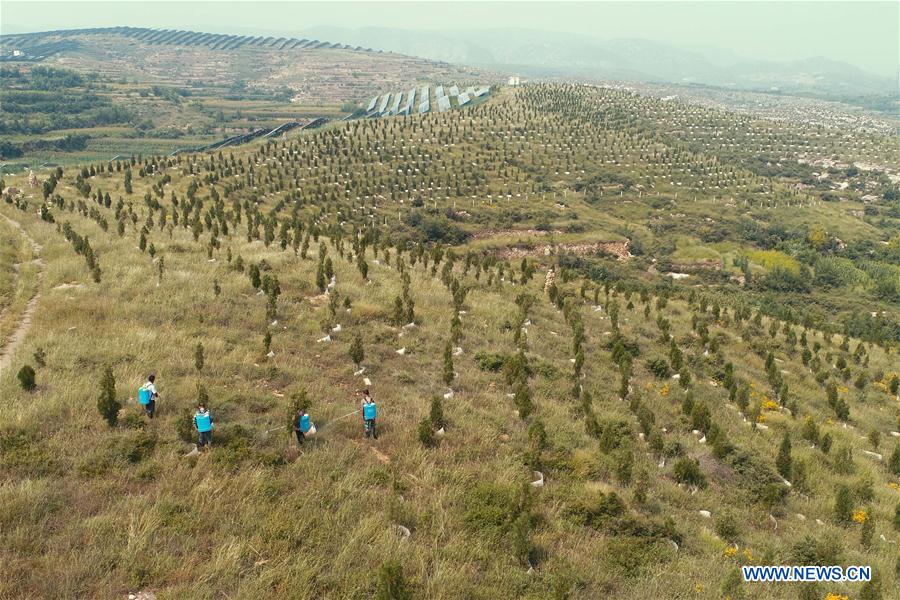The photograph depicts a vast expanse of gently rolling hills covered in dried grass with a mixture of dark green, human-height trees planted in lines at regular intervals, clearly the result of man-made efforts. The grassy fields stretch endlessly into the background, creating a patchwork of earthy brown and green hues. In the lower left corner of the image, four individuals with blue backpacks are seen walking along well-trodden paths, suggesting they may be attending to the trees. The lower right corner of the image features the website www.news.cn. As the hills undulate and curve, rows of trees appear spaced more densely towards the center and background of the image. Further back, solar panels or industrial structures can be seen, hinting at the presence of sustainable technology amidst this vast, cultivated landscape.